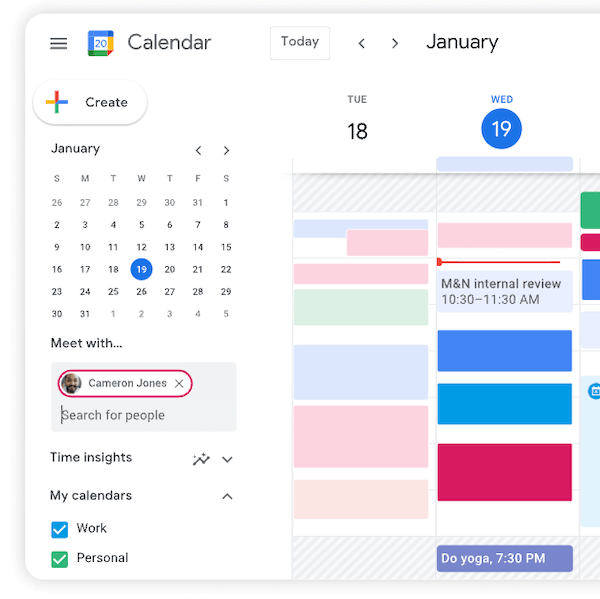In this image, we see a detailed view of the Google Calendar interface. At the top left corner, there's a hamburger menu icon. To its right, there's the Google Calendar logo, which is a square featuring layers of blue, green, yellow, and red colors, with the number "20" displayed in its center. Adjacent to the logo is the word "Calendar."

At the top center of the screen, there's a box with the word "Today," flanked by left and right arrows. To the right of these arrows is the label "January." 

Beneath this, on the left side, there's a bubble-shaped button that says "Create" along with a plus symbol on its left. Directly below this, there's a mini-calendar for January with the current date, the 19th, highlighted with a blue circle. 

Further down, there's a section labeled "Meet with" followed by a box containing the name "Cameron Jones," encased in an oval-shaped red outline. 

Below that, the section labeled "My Calendars" is present, displaying two categories: "Work" and "Personal." Each category has a checkbox on the left side, both with white check marks indicating they are selected.

In the central area of the screen, the dates "Tuesday 18th" and "Wednesday 19th" are visible in a vertical list. Notably, there's an event listed for "Do Yoga" scheduled at 7:30 PM on one of these dates.